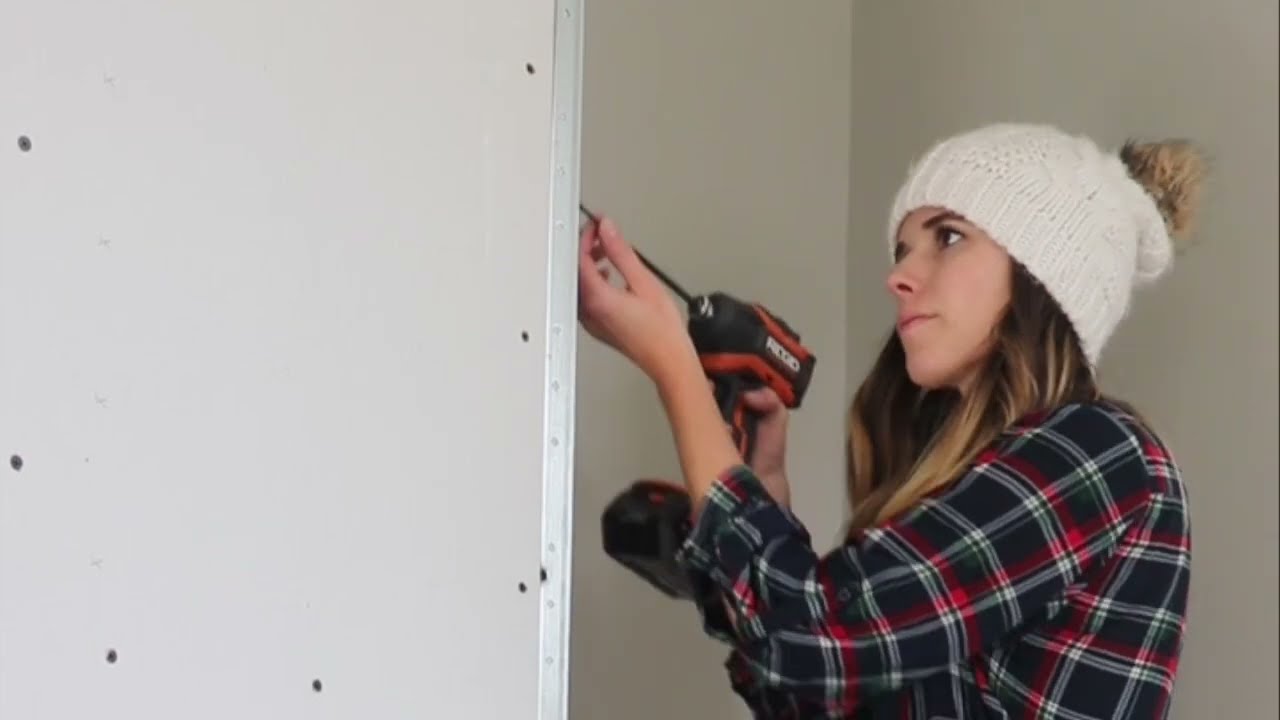The image captures a young woman, likely in her mid-twenties, engaged in a repair or construction task inside a house or building. She stands against a plain white wall that appears to be under construction, with visible screws and a thin metal strip at the corner. The left side of the image prominently displays this white wall with embedded screws, while the right side introduces a slightly darker beige wall.

The woman, who has long brown hair streaked with blonde, is dressed in a flannel shirt featuring a plaid pattern of red, green, and white. She accessorizes with a knitted white winter hat that has a fluffy, brown poofy ball at the top. With a focused expression, she uses a power drill to screw something into the wall. She holds the drill in her right hand, steadying it with her left hand close to the wall. The setting and her attire imply a casual but determined approach to her work, contributing to a detailed and authentic scene of do-it-yourself effort.